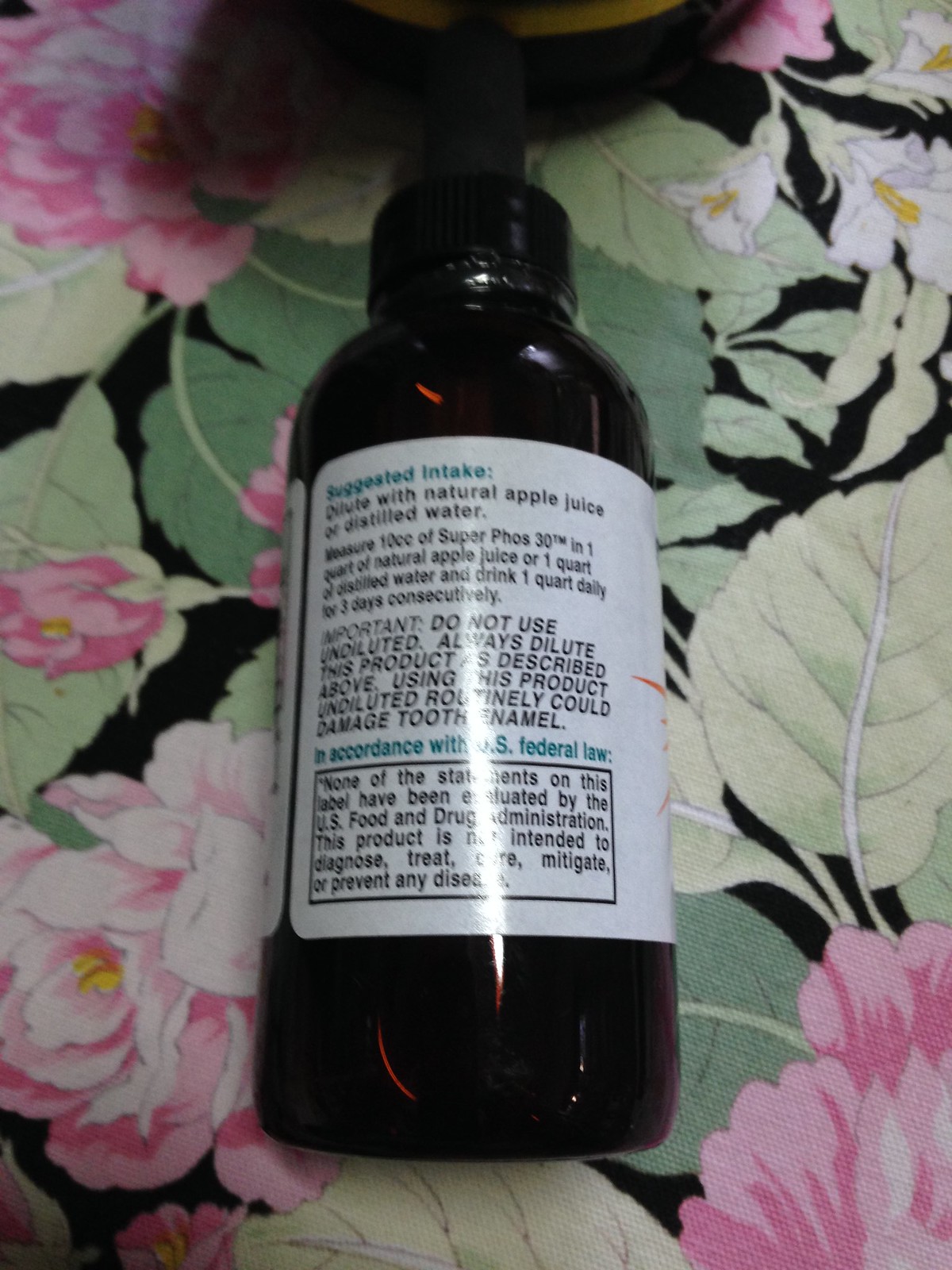The image depicts a small brown bottle with a black cap. The label on the back of the bottle provides detailed usage instructions for a product called "Super Fos 30." It advises users to measure 10 cc of the product and dilute it in 1 quart of natural apple juice or distilled water. The diluted mixture should be consumed daily, 1 quart per day, for three consecutive days. The label emphasizes the importance of dilution, warning that using the product undiluted can damage tooth enamel. Additionally, the label includes a disclaimer in compliance with U.S. federal law, stating that none of the claims have been evaluated by the U.S. Food and Drug Administration and that the product is not intended to diagnose, treat, cure, mitigate, or prevent any disease.